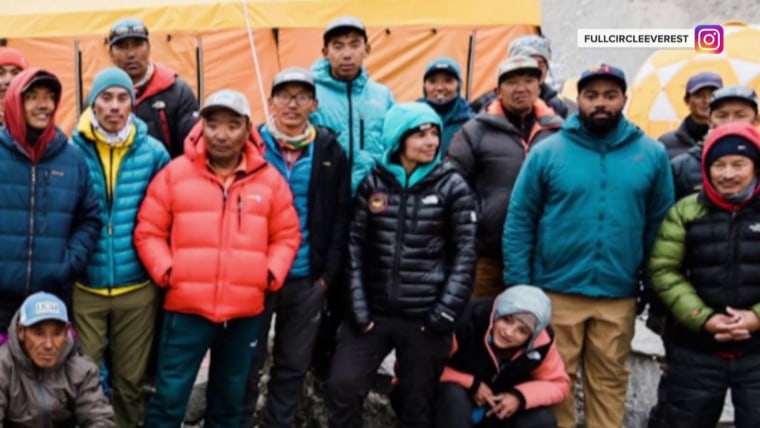In this vibrant and well-lit photograph, courtesy of the Full Circle Everest Instagram page, a diverse group of people collectively faces the camera, suggesting they might be climbers or guides associated with a Mount Everest expedition. They are dressed in a variety of brightly colored outdoor attire, including heavy jackets and bubble vests, in shades ranging from blue to dark blue, green, orange, black, and olive green, with everyone also sporting various types of hats. Notably, the group appears to be in a camping area, as evidenced by the orange, yellow, and white tents visible in the background. The group includes both men and women, although men are more prominently featured. The scene is set against a backdrop that includes both clustered tents and what might be a building. The overall clarity of the image is high, showcasing each individual's gear and expressions in detail, under plenty of natural lighting. The "Full Circle Everest" logo in the top right corner emphasizes the likely adventurous and challenging nature of their endeavor.